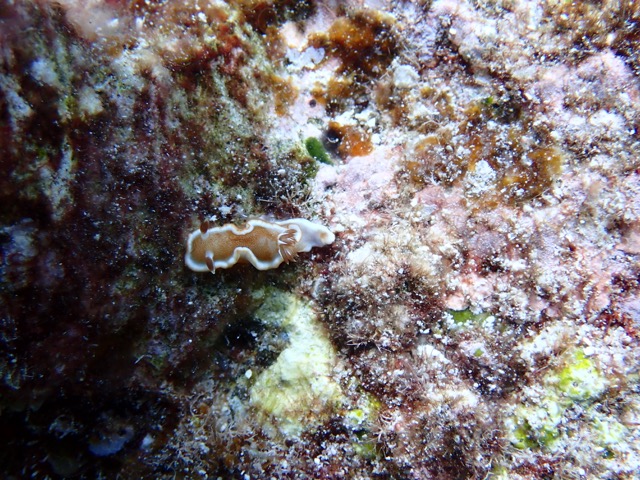The image showcases the floor of an ocean, featuring a variety of textures and organisms. Dominating the center is a squiggly, wet creature with a beige hue and white accents. The right side is characterized by a patch of fuzzy mold or bacterial growth, displaying an array of colors including white, light pink, neon green, dark brown, amber, and beige specks. This intricate and multicolored mold creates an almost surreal appearance. In contrast, the left side of the image is notably darker, shaded in maroon and brown tones, providing a stark juxtaposition to the vibrant right side. The scene captures the rich and diverse ecosystem found on the ocean floor, highlighting the intricate interplay between marine life and its environment, though its appearance might be considered unsettling to some.